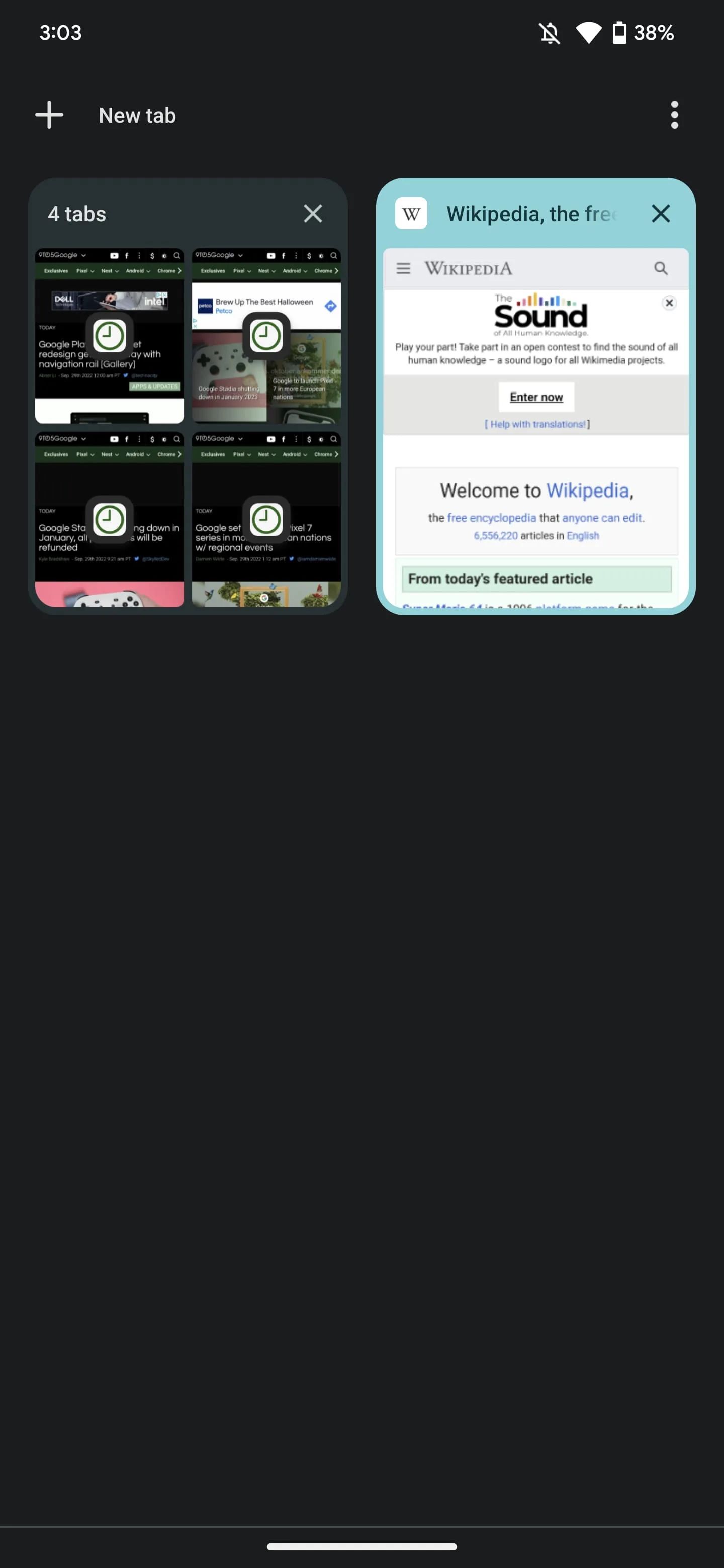In the top right corner of the screen, there are icons indicating a 303 notification, Wi-Fi signal strength, and battery status. Below these icons, the browser displays four tabs, with the first one labeled "New Tab" and the second one showing the Wikipedia page, where the word "sound" is clearly visible. The other two tabs are too small to discern any specific details. The Wikipedia tab is currently active, and the page displays a welcoming message. The entire background of the screen is black, with a distinct white line running across the bottom.